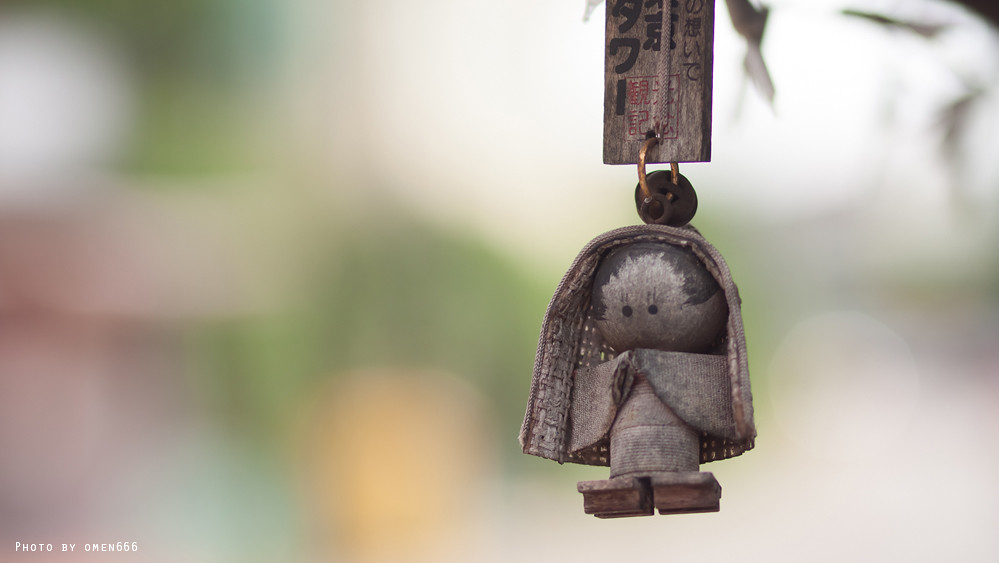The daytime photograph features a charming, intricately detailed wooden figurine set against a heavily blurred backdrop of green, with hints of pink, yellow, and white in the far right background. Prominently displayed in the foreground towards the right, the figurine, resembling a small nun or bride with a round face marked by two simple eyes, is adorned with what appears to be traditional Japanese attire. It has a cylindrical body with robe-like sleeves and geisha shoes, while a rectangular wooden plaque with black Japanese or Chinese writing is attached above it by a copper ring. The figure's head, a carved wooden ball, sports a shawl-like covering, giving the impression of tied-back hair. Adding a final touch of authenticity, the bottom left-hand corner of the image bears the white lettering, "Photo by Ullman666."